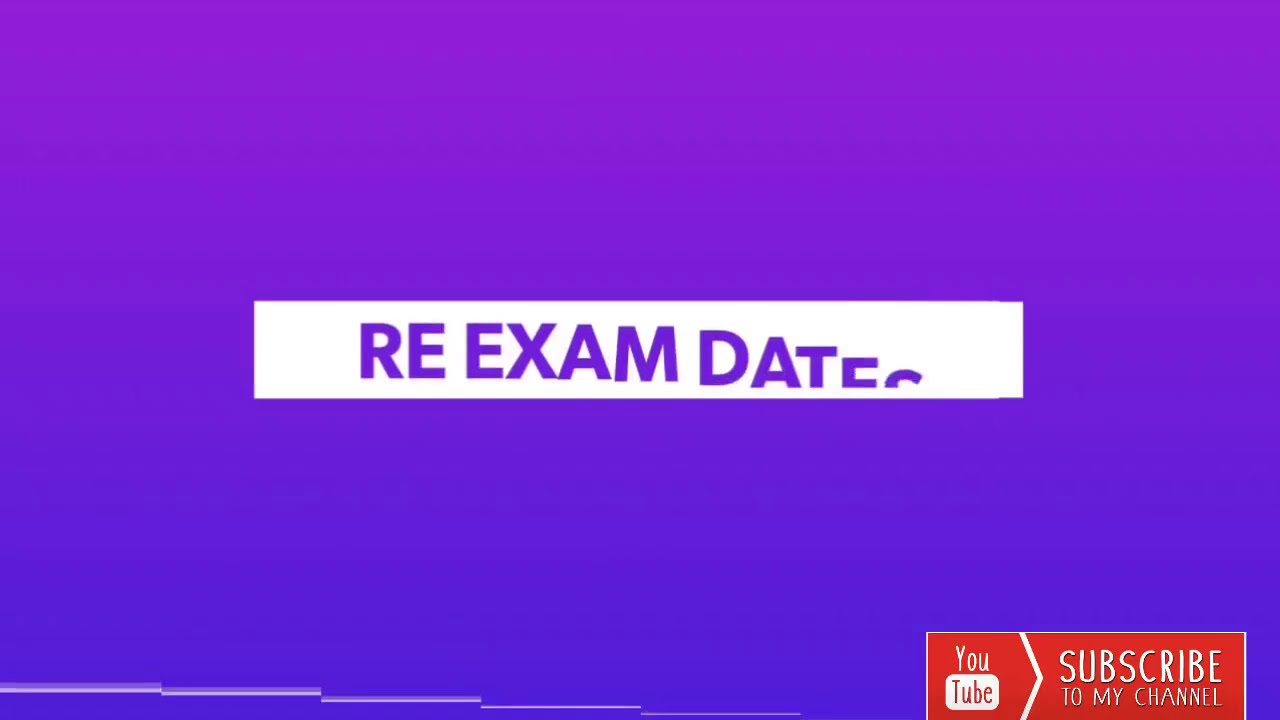This digital text image features a minimalist graphic design with a primarily purple gradient background, transitioning from a light grape purple at the top to a deep purple at the bottom. Centered within the image is a prominent white strip containing the text "RE-EXAM DATES" in blue capital letters. Notably, the letters in the word "DATES" descend stepwise, with "E" and "S" almost completely hidden.

Additionally, the lower left side of the image displays a series of white lines arranged to mimic steps. On the lower right corner, there's a red rectangle featuring the YouTube icon accompanied by the text "SUBSCRIBE TO MY CHANNEL" in white capital letters. This text and icon capture attention against the gradient background, completing the visual design.